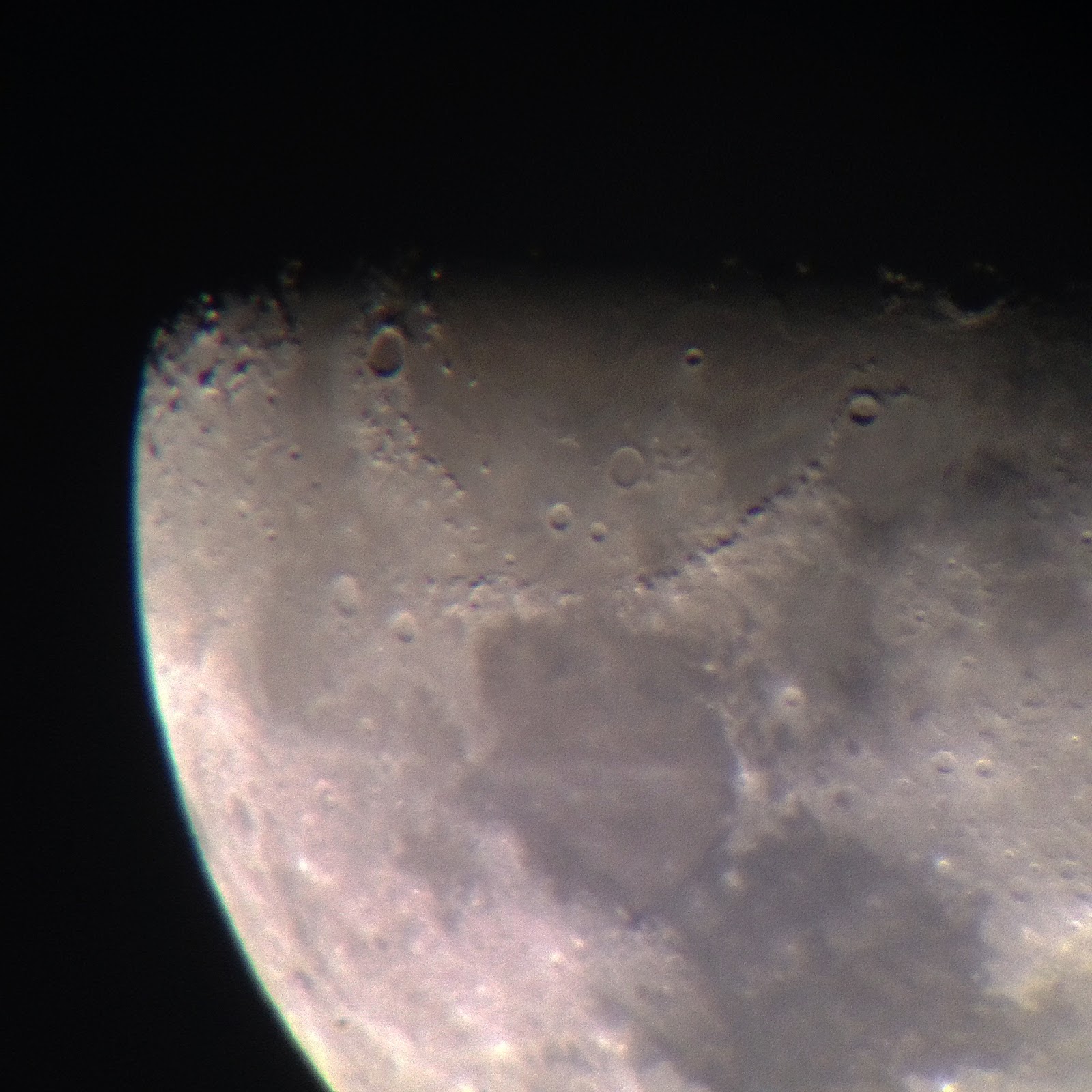This image appears to be a close-up of the moon's surface, displayed in large square format with no border. The upper part and the left side of the image are predominantly a solid black. The left side also reveals the rounded edge of the moon, transitioning from dark gray to light gray and white along this curved boundary. The photo, which seems to focus on the lower quarter of the moon, features numerous small, circular craters scattered across the surface. Toward the top of the image, the craters become more prominent and densely packed. Additionally, the lower right-center of the photo shows two particularly dark and deep craters. The image, appearing in black and white, suggests substantial illumination in the lower left part, possibly due to sunlight hitting it directly. The varying shades of gray and the contrasting black areas add depth and emphasize the intricate details of the lunar landscape.